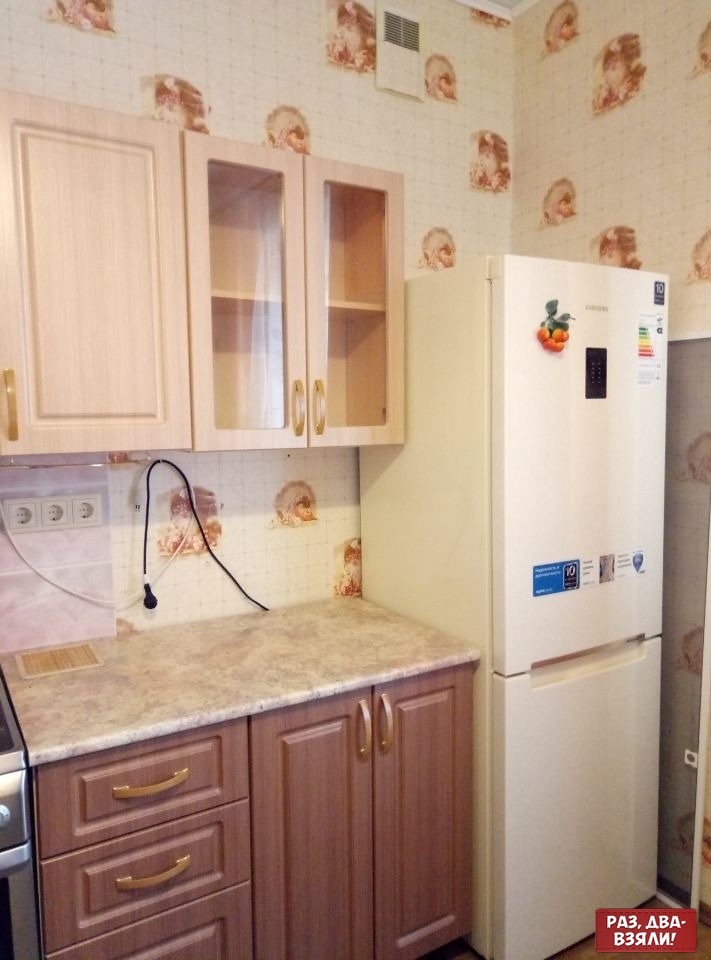This photograph captures the corner of a kitchen featuring distinct elements and details. The walls are adorned with cream-colored tiles that have a peculiar, repeating pattern resembling smeared blood or fossil drawings, adding an unusual artistic touch to the space. In the corner stands a white refrigerator-freezer combo, with the fridge above the freezer. The refrigerator is adorned with stickers, including one with a rainbow design and another that looks like a fake fruit magnet. The center of the refrigerator has a black square, while a blue rectangle can be seen towards the bottom. Below the white-tiled walls is a countertop made from an imitation marble surface, bordered with dark brown cabinetry featuring gold accents on the handles. Above the countertop, lighter brown cupboards fitted with the same gold hardware provide additional storage. An electrical outlet trinity punctuates the tiled wall, and towards the bottom right of the image, a red square sign with white text, possibly in Russian, is visible, adding a pop of color to the predominantly neutral palette. On the left side of the image, a sliver of a stainless steel range peeks into view, completing this meticulously detailed kitchen scene.